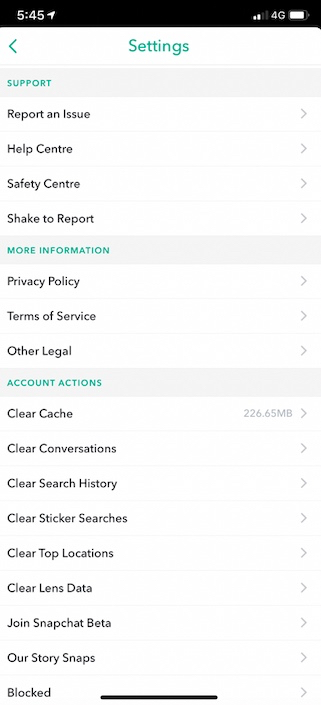The image depicts the settings page of the Snapchat app on a smartphone. At the top of the screen, there's a black navigation bar showing the time as 5:45 on the left side and a battery indicator on the right, which appears to be 95-97% full. 

The main settings page has a white background with section titles in green text and specific options in black text. The page's title, "Settings," is prominently displayed at the top in green. 

The first section, labeled "Support," includes several drop-down menus: 
- Report an Issue
- Help Center
- Safety Center
- Check to Report

Following that, the "More Information" section also contains several options:
- Privacy Policy
- Terms of Service
- Other Legal

The last section, "Account Details," has multiple drop-down menu options including:
- Clear Cache (showing 226.65 MB on the right)
- Clear Conversations
- Clear Search History
- Clear Sticker Searches
- Clear Top Locations
- Clear Lens Data
- Join Snapchat Beta
- Our Story Snaps
- Blocked

This detailed image captures the comprehensive settings menu of the Snapchat application, highlighting the various categories and options available for user customization and support.